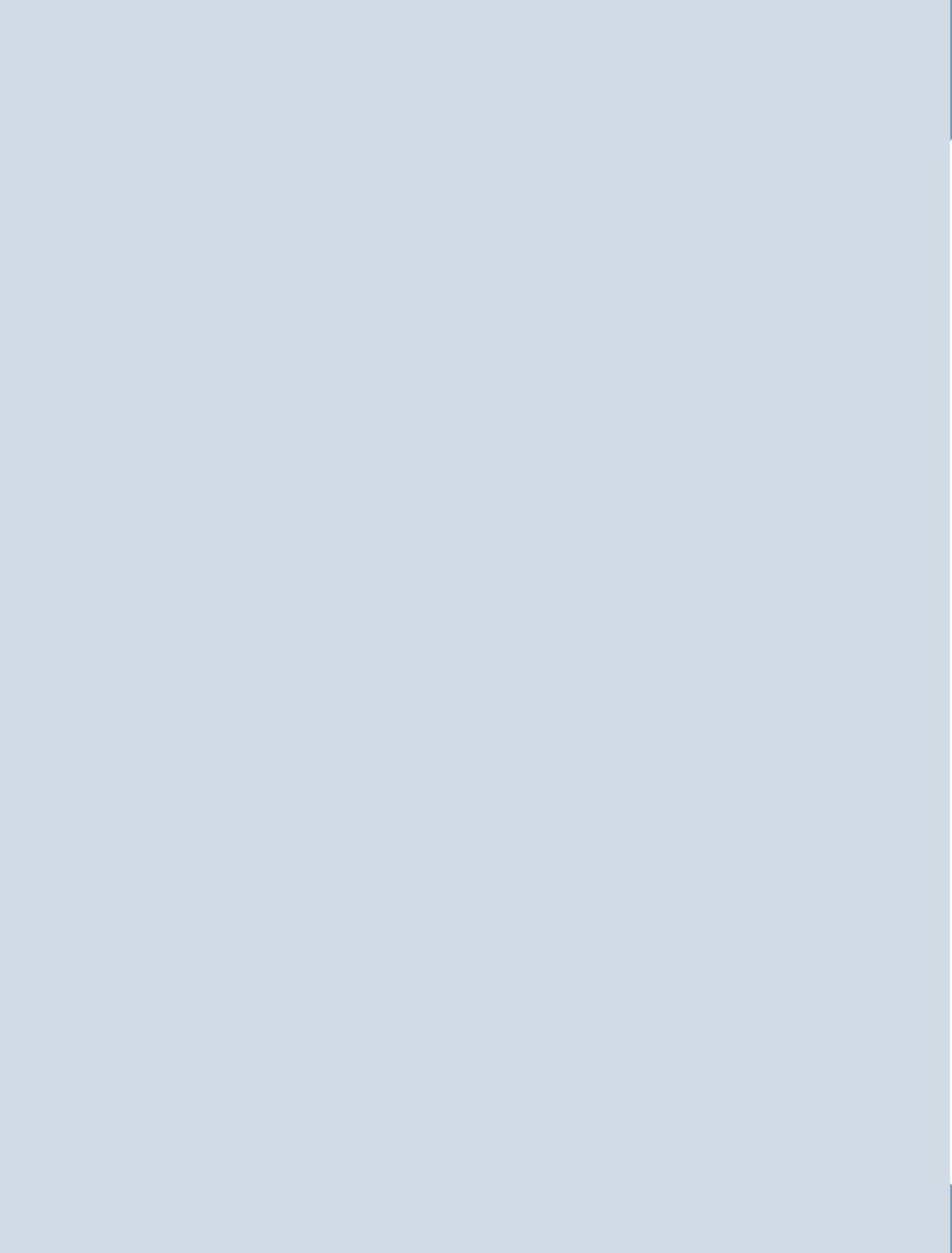The image is a vertical composition, approximately 50% taller than it is wide. Dominated by shades of gray with a hint of blue, the overall color palette is a muted, slightly darker gray with subtle blue undertones, creating a serene and understated aesthetic. 

In the upper right corner, around 15% down from the top edge, is a narrow navy blue line that runs vertically along the right side. A similar navy blue line can be found at the bottom of the image, extending vertically along the right edge, covering roughly 8% of the image's total height. These dark blue lines add a subtle contrast to the predominantly gray tones, creating a minimalist yet intriguing visual composition.